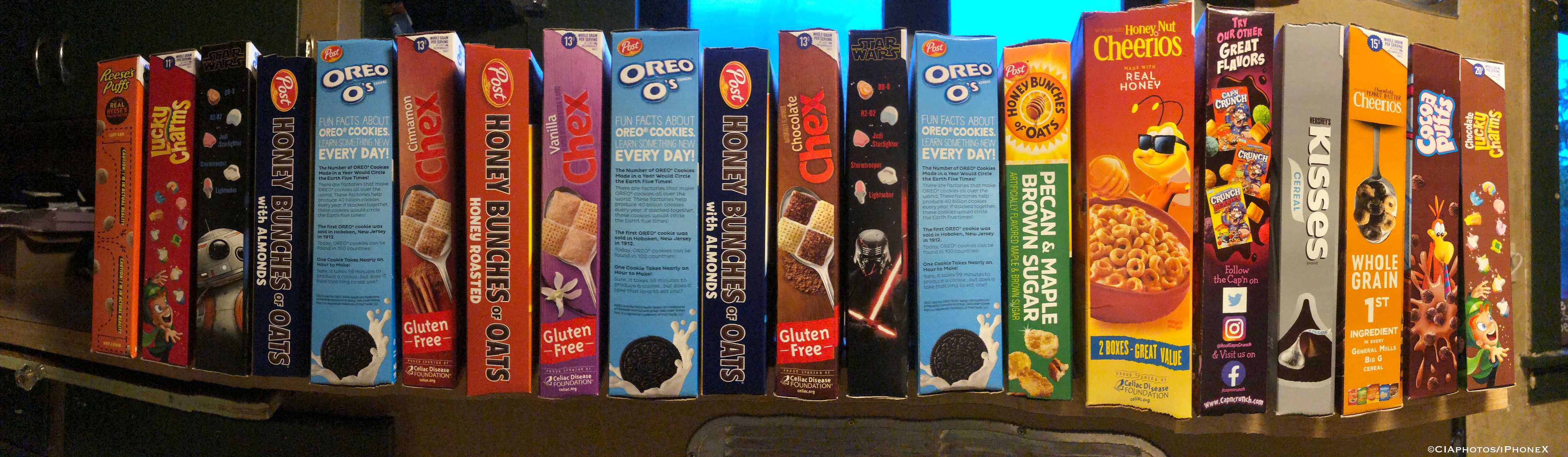This is a color photograph showcasing a well-organized brown shelf brimming with an array of food packets that at first glance might be mistaken for books. The shelf, captured in a long, narrow frame, prominently features a neat lineup of vibrant packages. Among them, three blue boxes of Oreos are distinguishable, each adorned with an enticing image of the cookies. A cheerful red and yellow Cheerios box stands out amidst the collection. Additionally, a product labelled "Kisses" is noticeable among various other cereal and food boxes in shades of black, red, blue, and multiple other colors. Some of these items are duplicated, indicating popular or frequently used products. Behind the shelf, towards the middle, a window can be seen, framed by a pale blue structure with a central pane, allowing light to filter in. To the right, part of a beige wall is visible, with the edge of another window hinting at the continuation of the room's layout.